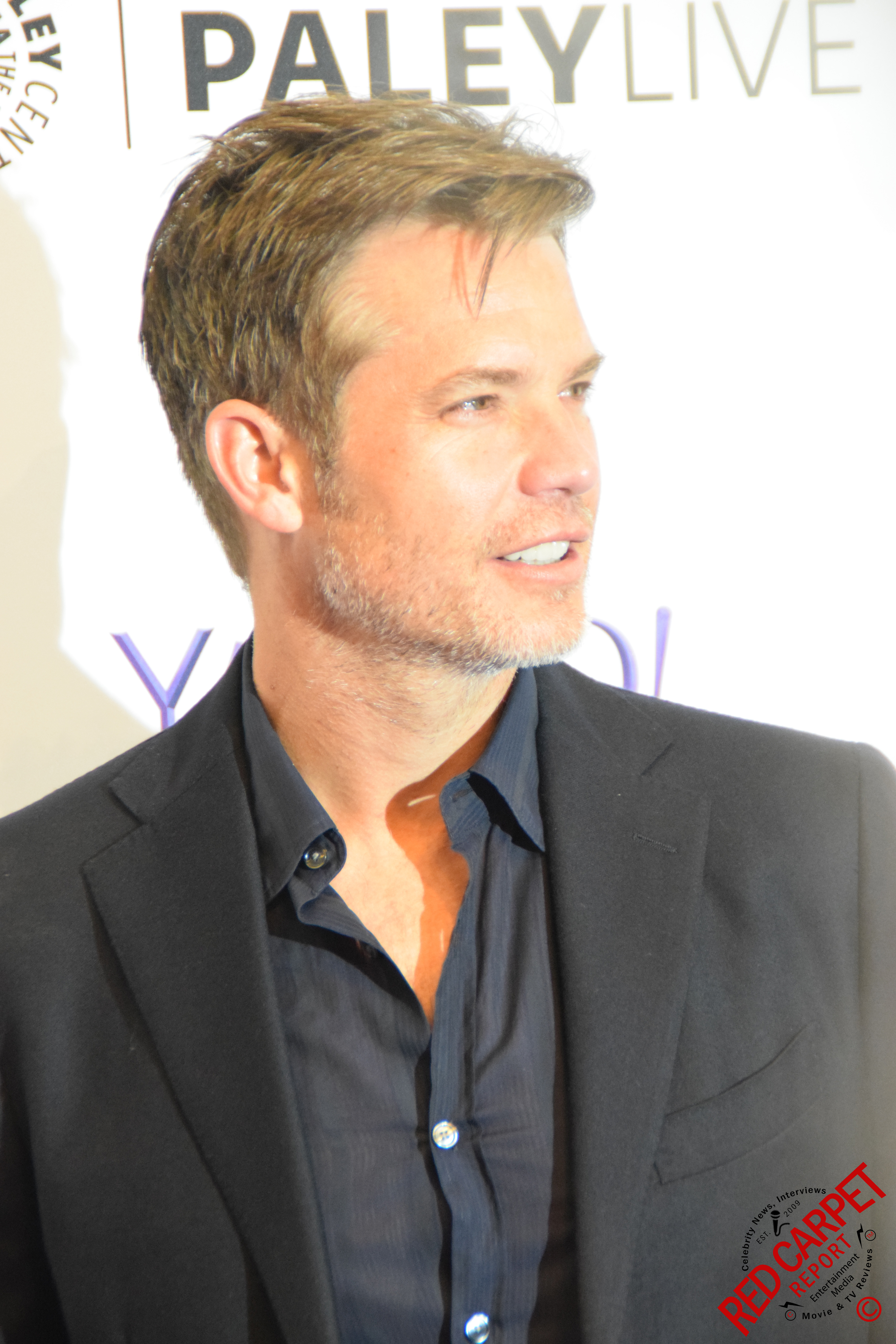In this detailed photo, actor Timothy Olyphant is featured in a side profile, turned slightly to his right but gazing towards his left. He has short, sandy blonde hair with hints of gray and wears a short, grayish beard styled like a goatee. He is partially smiling, his teeth subtly visible. Clad in a dark suit jacket—described variably as gray or black due to the reflective light—and a darker button-up shirt, Olyphant stands against a stark white backdrop. 

This backdrop features the words "Pally Live," with "Pally" bold and a purple "Y," creating a significant shadow behind him due to a bright light. In the bottom right corner of the image, the red diagonal text "Red Carpet" is encircled by additional text reading "Celebrity News, Interview, Established 2009, Red Carpet Report, Entertainment Media, Movie and TV Reviews," with a small red copyright symbol and a microphone icon marking the center of the circle.